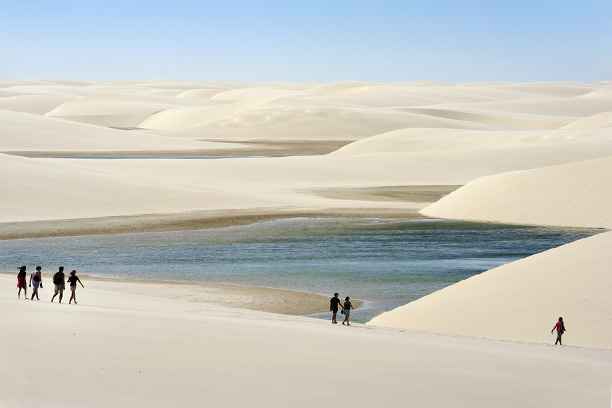Set amidst a vast landscape of tan sand dunes, this striking image captures a serene oasis at its heart—a diamond-shaped body of blue water glimmering under the bright blue sky. The picturesque sand dunes roll gently towards the horizon, forming an undulating backdrop enveloping the tranquil water. Scattered across the foreground are seven people: a group of four on the bottom left, including three boys in black, white, and gray shirts, accompanied by a girl in a red dress; closer to the water in the middle, a couple—possibly young adults—walks together, both in casual shorts and short sleeves; and off to the bottom right, a solitary woman clad in jeans and a blue garment strolls thoughtfully. These individuals, with varied attire and body language, add dynamic life to the otherwise still and arid desert scene, moving either towards the refreshing water or further into the desert expanse.